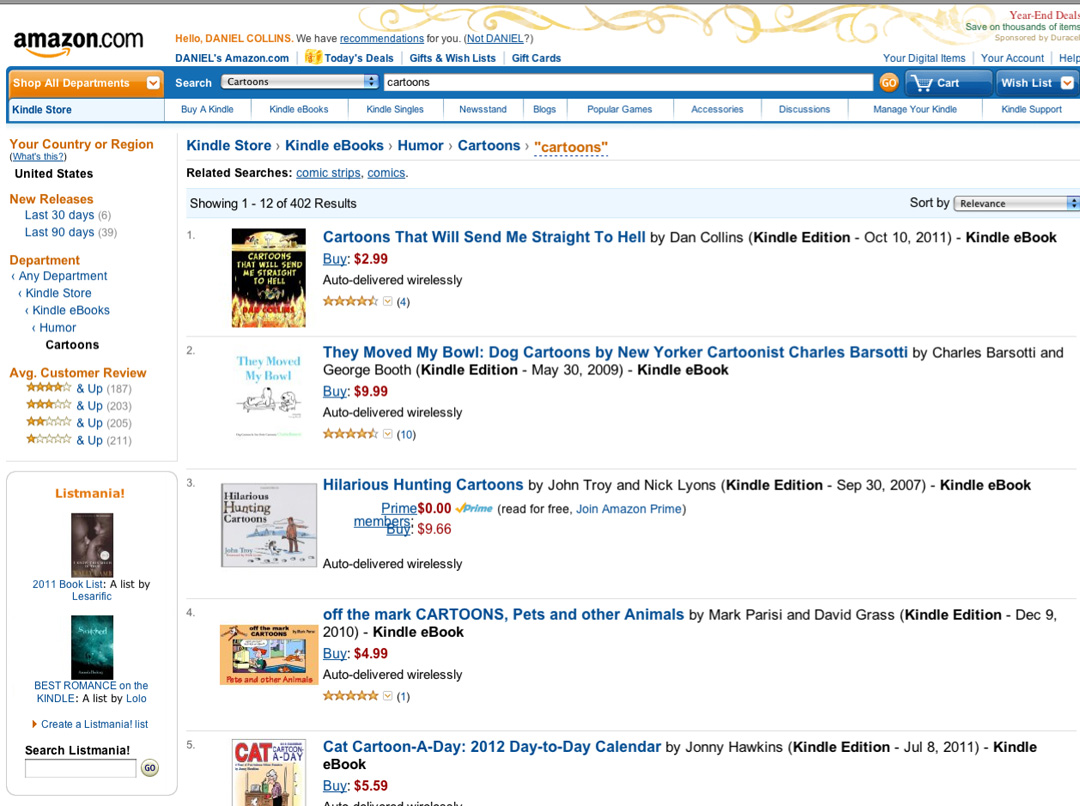This is a detailed screenshot of the Amazon.com homepage. In the top-left corner, the Amazon logo is prominently displayed with its signature orange arrow pointing from the "A" to the "Z." Next to the logo, "Amazon.com" is written in orange font. Below this, the greeting "Hello, Daniel Collins" is visible, accompanied by a blue clickable link prompting recommendations. This is followed by a parenthetical, clickable link that reads "Not Daniel?"

Below the greeting, the navigation options "Daniel's Amazon.com", "Today's Deals," "Gifts & Wish Lists," and "Gift Cards" are displayed. Beneath this, a blue navigation bar features an orange button on the left labeled "Shop All Departments." The navigation bar has "Search" in white font with a drop-down menu currently set to "Cartoons." A search bar also labeled "Cartoons" is present, followed by an orange circular button marked "Go," an option for the shopping cart, and a drop-down for the wish list.

Further down, the Kindle store section is visible within the navigation bar, listing options such as "Buy a Kindle," "Kindle eBooks," "Kindle Singles," "Newsstand," "Blogs," "Popular Games," "Accessories," "Discussions," "Manage Your Kindle," and "Kindle Support."

The main content area displays search results for cartoons, featuring various books suggested based on the search query. The left-hand side of the page contains options to filter the results, while the right-hand side offers sorting options.